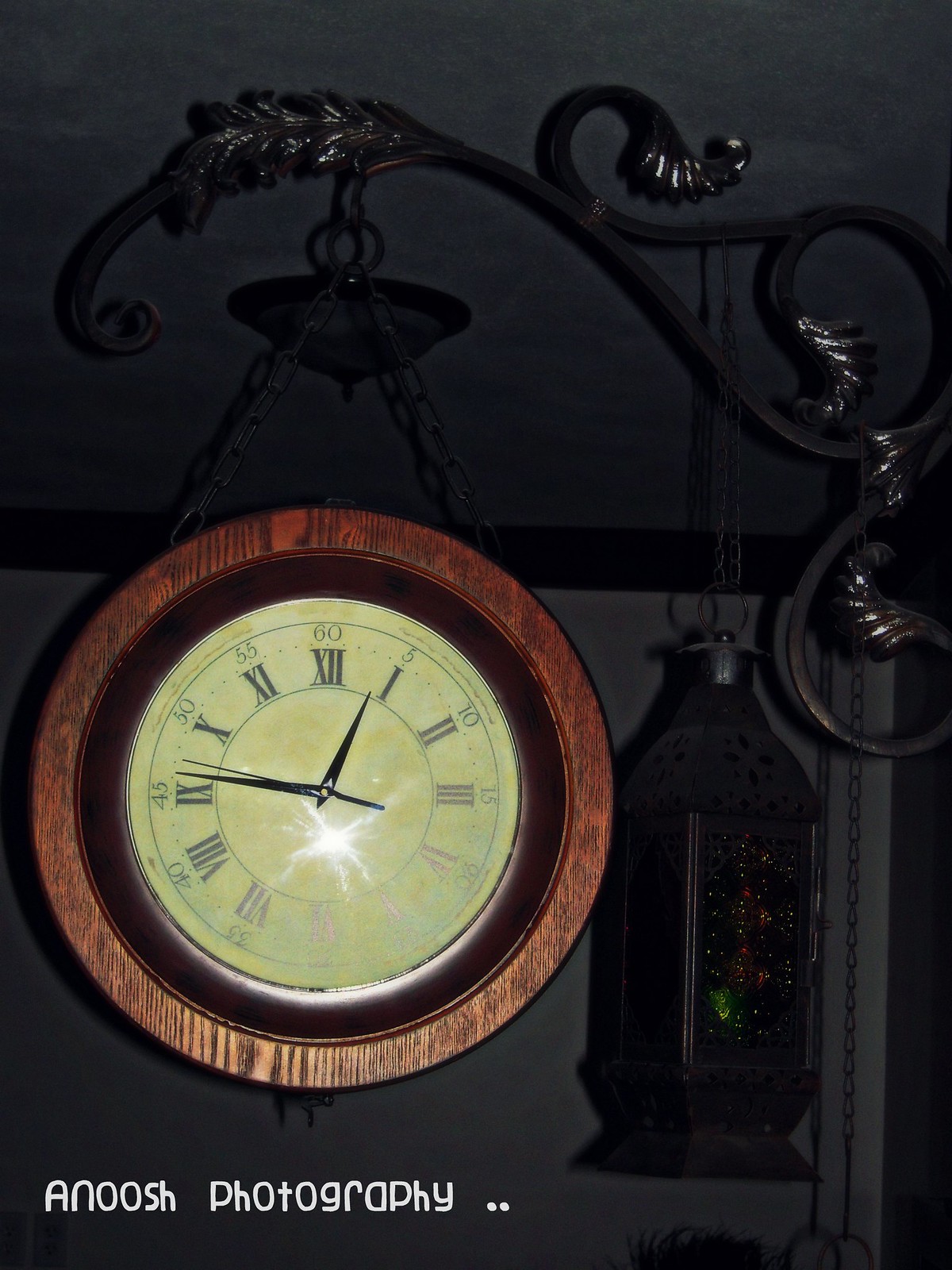The image depicts a vintage clock suspended from an ornamental black metal bracket mounted on a side wall. The clock, framed in a dark wood-like material, hangs downwards supported by black chains attached to the ornate holder. Its face is a pale, whitish-yellow hue and features Roman numerals paired with an outer circle marking seconds at intervals of 5, 10, 15, and so on. At the bottom left corner of the clock face, the text "Anoush Photography" is printed in white, accompanied by two small white dots.

Adjacent to the clock, also hanging from the same ornamental structure via a black chain, is a small lantern with a distinctive reddish-greenish glow emanating from within. The backdrop of the scene is shrouded in darkness, with both the ceiling and walls appearing black, indicating that the setting is inside a dimly lit room.